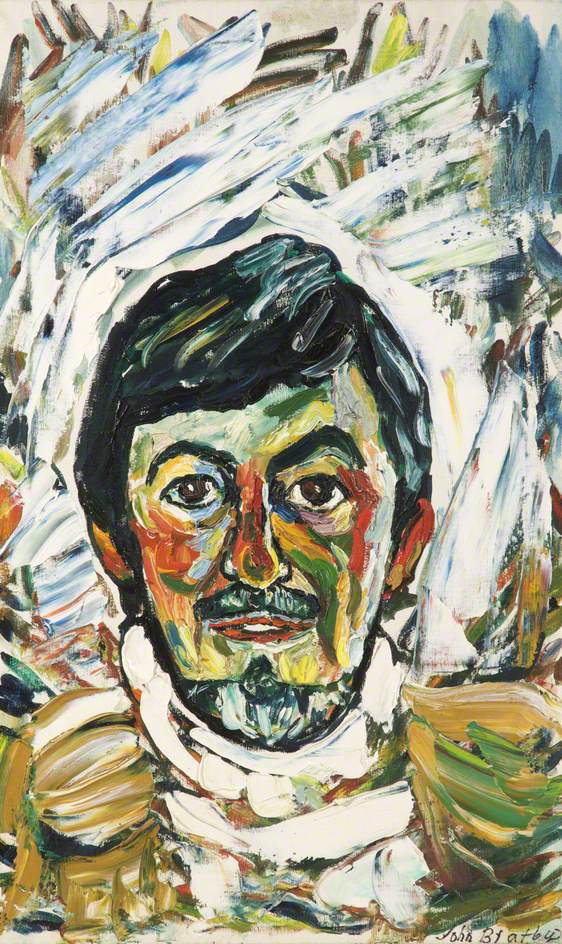This contemporary portrait painting features a man facing forward, centered within a vertical rectangle canvas. His short, black hair and prominent, dark black eyebrows frame his expressive large black eyes. The man sports a black mustache and a black goatee, with a very subtle smile playing on his lips, which are painted red. His face is a vibrant blend of bluish, brown, yellow, and green hues, with thick, broad brushstrokes defining the contours and highlights of his cheeks, forehead, and jawline, making the features jump out even though the style remains distinctly abstract. The man's neck is accented with thick bands of pure white, and his shoulders, though blending into the background, reveal a brown jacket over a white shirt. Surrounding the portrait, the background is a chaotic yet harmonious mix of heavy brushstrokes in white, with patches of blue, yellow, gray, tan, and green, adding to the modern, textured feel of the piece. The raw, unrendered brushstrokes emphasize the boldness and dynamism of this striking artwork.